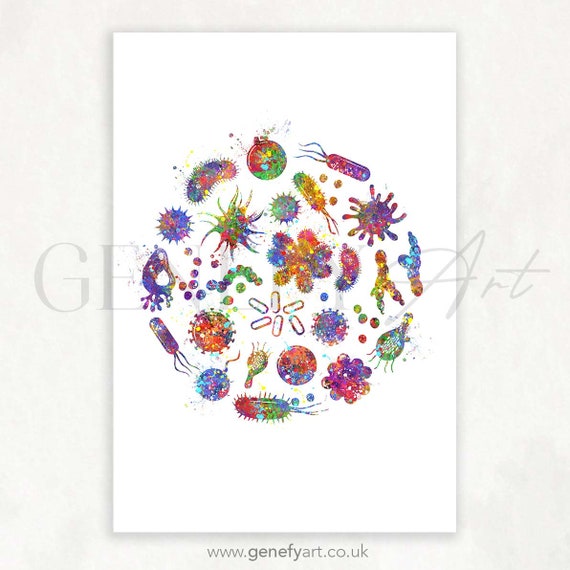This image showcases a highly detailed product advertisement for a piece of vibrant artwork by Genify Art. The central feature of the artwork is a vertical print on white paper placed on an off-white surface. This print depicts a circular arrangement of neon-colored illustrations of various microorganisms, including amoebae, bacteria, protozoa, and viruses, reminiscent of a tie-dye or Lisa Frank style color palette. Each microorganism is intricately designed, ranging in shape from rod-like forms with tails to circular entities adorned with spikes. The illustrations fill the entire circle against a white background, and the vivid hues create a striking visual effect. A watermark reading "Genify Art" spans across the center of the artwork, while the website "www.genifyart.co.uk" is displayed at the bottom of the image.